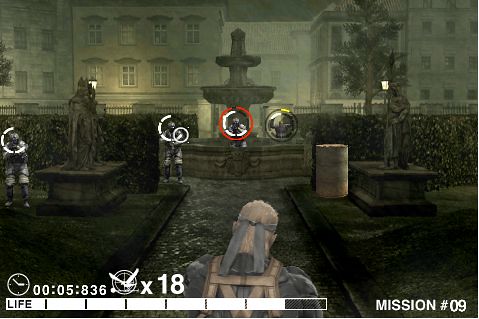The image is a screen capture from a video game. At the bottom of the screen, there is a white play timer and a life bar indicating the player's health. The text "Mission Number Nine" is displayed in white font. The scene is set in front of an elaborate mansion during the nighttime. 

In the foreground, a character wearing a vest, dark shirt, and gray headband stands facing armed soldiers. The soldiers are positioned around a stone water fountain in front of the mansion. Two stone statues are visible on either side of the yard. One soldier is crouched within the fountain, while two others are on the right side of the screen. One soldier has a red circle around him, while two have white circles. Behind the fountain, there is a blurry figure partially encircled by a yellow circle, making it difficult to identify. Light posts are scattered around the mansion's exterior, casting reflections on its windows.